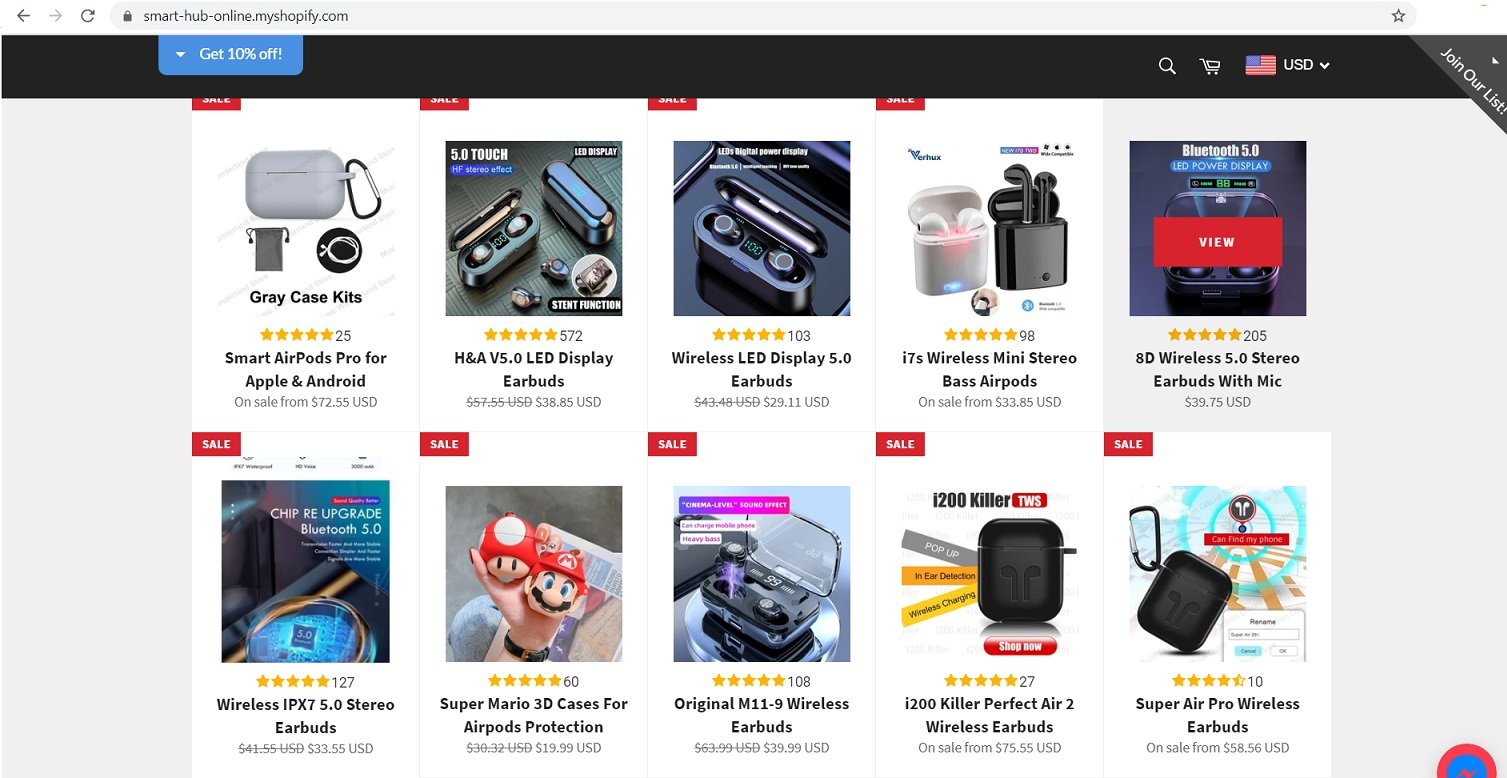An image showcasing a drop-shipping storefront on Shopify’s smarthubonline.myshopify.com platform. The website features a clean, light gray background with a white product display area. 

**Header Details:**
- In the upper left corner, a prominent blue button with white text offers "Get 10% Off."
- The upper right corner features a magnifying glass icon for search, a currency selector marked by "USD" and accompanied by a flag, and a call-to-action prompt to "Join our list."

**Product Display:**
- The storefront displays two rows of products, with each row showcasing six items.
- The upper left product is labeled as "Smart AirPods Pro for Apple and Android."
- The remaining items consist mainly of various earbuds and phone accessories, indicating a focus on audio technology and mobile peripheral devices.

The layout and the type of items suggest that this might be a drop-shipping store, aiming to offer popular tech accessories to a wide audience without maintaining physical inventory.